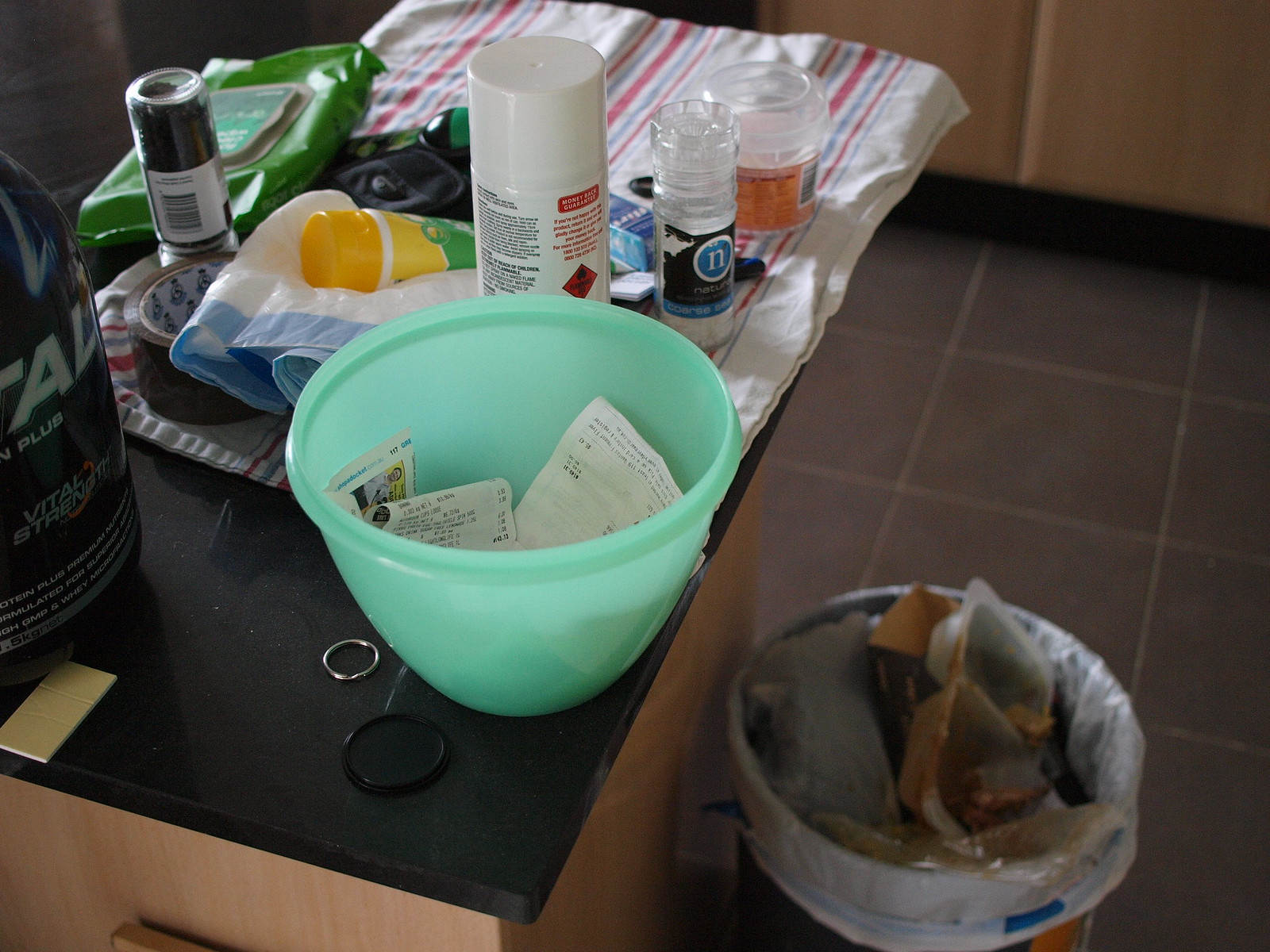On a light brown wooden kitchen cabinet with a black granite countertop, a disorganized array of items can be seen. There are several seasoning containers, with the black cap of one missing. A green bowl, seemingly filled with receipts, adds a touch of color. The surface appears cluttered with loose items, including what looks like a partially folded baby blanket from a hospital, which has various seasonings and other small items scattered on top. Nearby, a pack of green wipes—likely Lysol disinfecting wipes—sits behind the blanket. The scene extends down to the dark gray tiled floor, where a nearly full trash bin is visible, indicating a need for emptying. The overall view portrays an everyday kitchen scene with a touch of disorder.